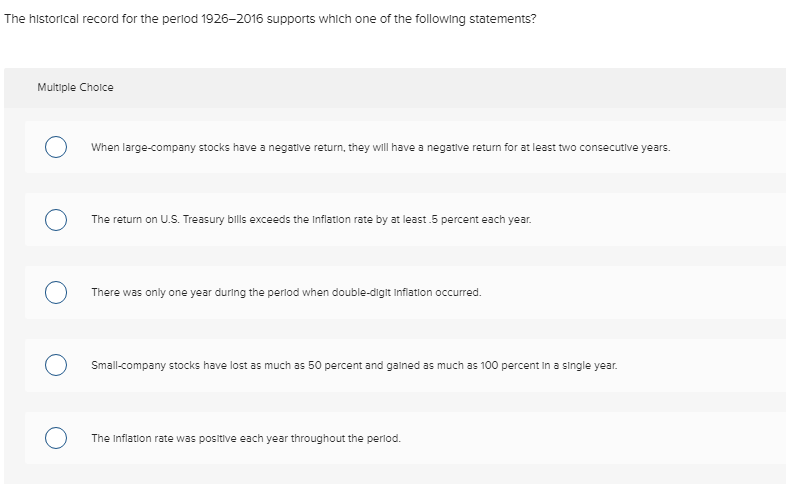A historical record spanning from 1926 to 2016 is displayed, supporting several statements for a multiple-choice question. The question is located in a gray box. 

The black text within the box reads "Multiple Choice," and below it are five answer options with corresponding radio buttons to select the correct response. The choices are:

1. When a large company's stocks have a negative return, they continue to have a negative return for at least two consecutive years.
2. The return on U.S. Treasury bills exceeds the inflation rate by at least five percent, or 0.5% each year.
3. There was only one year during the period when double-digit inflation occurred.
4. Small company stocks have experienced losses up to 50%, and gains as much as 100% in a single year.
5. The inflation rate was positive each year throughout the period.

The historical data itself is placed at the top of the area, detached from the multiple-choice section, surrounded by a white background. The multiple-choice options are formatted with black text within a gray shaded box. The answer bubbles, situated to the left of each statement, feature a light, thin blue border.